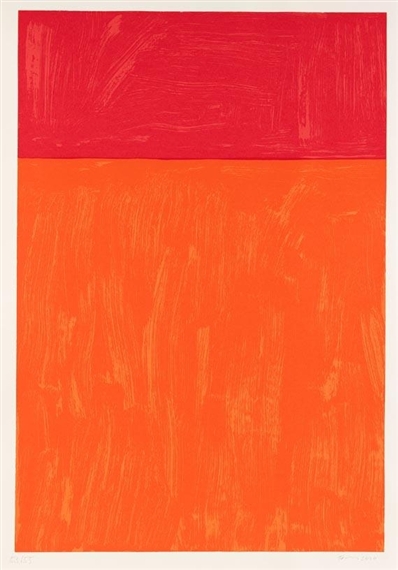This image depicts a modern painting characterized by simplicity and the expressive use of two primary colors: orange and dark red. The rectangular artwork is predominantly orange, covering approximately three-quarters of the canvas from bottom to top. This brilliant, bold orange appears to be applied with dynamic vertical brushstrokes and contains visible streaks of a lighter shade of orange, contributing to a textured, layered appearance.

The top quarter of the painting shifts to dark red, deliberately rich and deep in hue. Similar to the orange section, the dark red area also features vertical streaks, some slightly bent towards the right, enhancing the sense of movement and intensity within the piece.

The overall structure of the image loosely resembles the design of a cigarette pack, with the red section reminiscent of the part you'd pull off and the bulk of the orange akin to the body of the pack. The artwork is bordered by a light-colored frame, possibly white or tannish, which provides a subtle contrast to the vibrant colors within.

Notably, the application of paint appears somewhat uneven, with drips and runs visible throughout both color blocks, suggesting the use of a single coat that adds to the raw, emotional impact of the work. This stylistic choice, combined with the bold color palette, evokes a sense of emotional intensity, potentially reflecting the artist's mood during its creation.